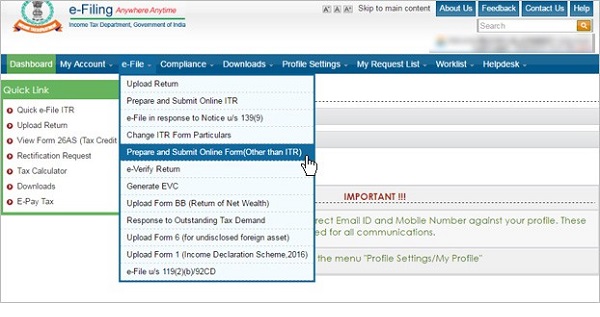A user is actively engaging with a dated e-filing website, potentially from the mid-2000s. The webpage features an option labeled "Prepare and Submit Online Form," with the user's cursor hovering over it, indicating their intention to proceed. Despite the mundane appearance, the site facilitates form submissions from any location at any time, underscoring its once-innovative functionality.